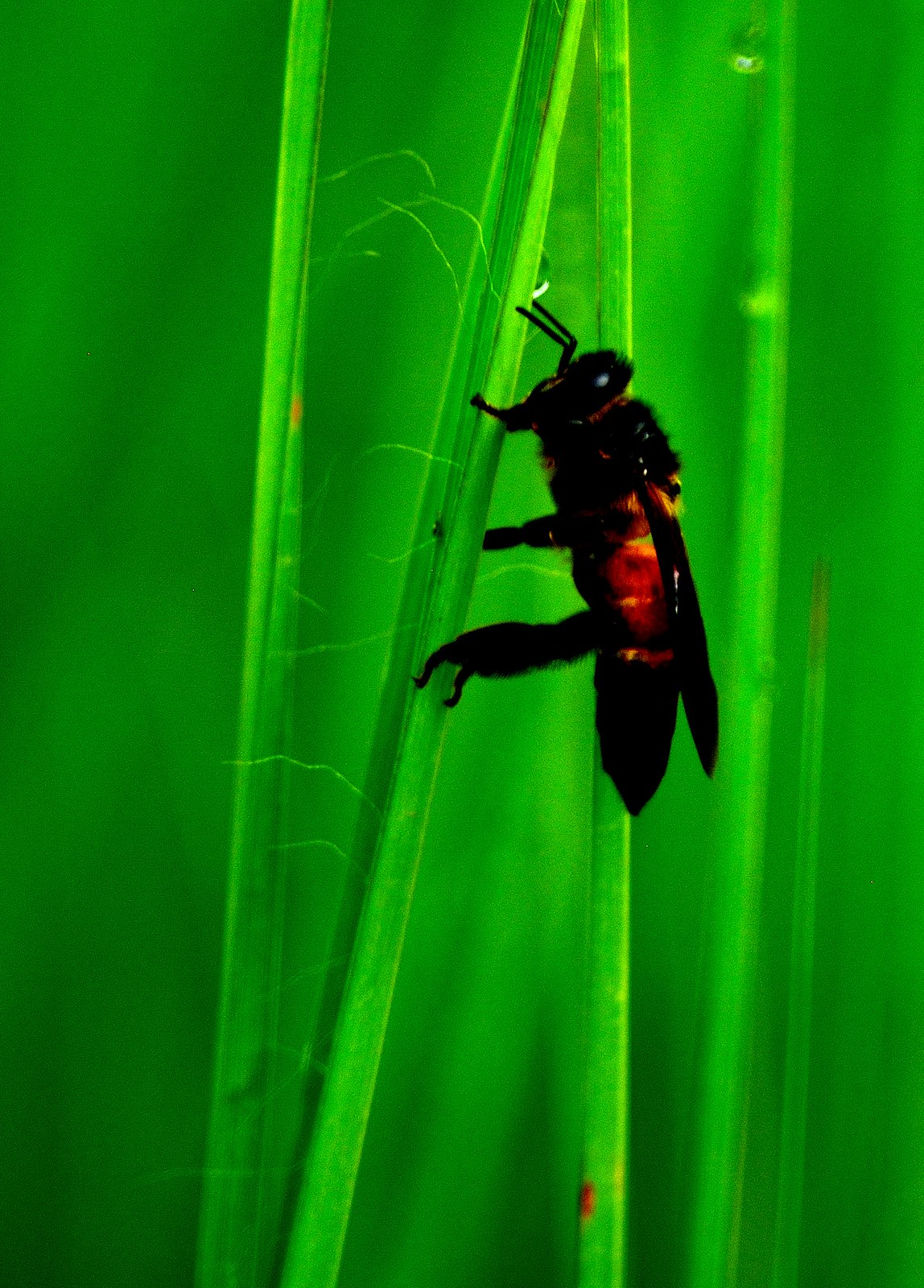In this captivating nature photo, a small, predominantly black insect—likely a wasp—clings vertically to a bright green blade of grass. Set against a vibrant, leafy green background comprising tall plant leaves or grasses, the insect is positioned slightly to the right of the image’s center. The wasp features a black body, legs, antennae, and wings, with a striking deep orange or dark red segment in the middle of its body. Its oval-shaped head extends two antennae outward, and it appears to be either climbing or feeding on the stem. The close-up perspective of the photo highlights the intricate details of the insect while emphasizing the lush, natural environment, offering a stunning and detailed glimpse of this small creature in its outdoor habitat.